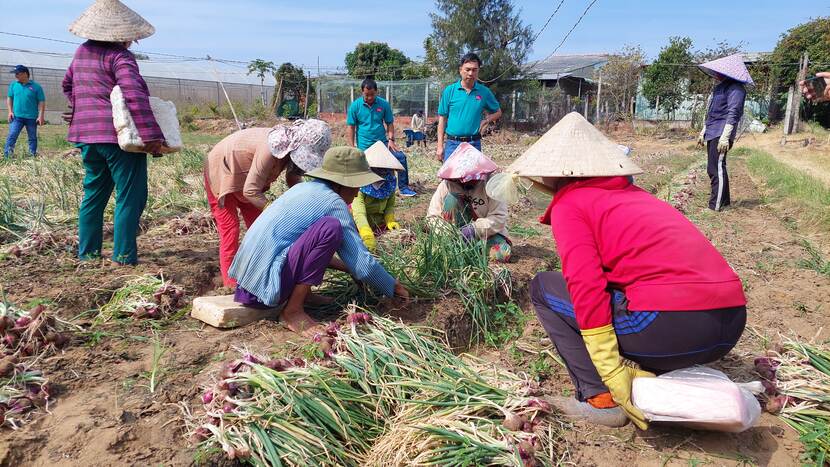In this image, a group of seven female workers is seen harvesting green onions or scallions on what appears to be a farm. The women are dressed in casual, long-sleeve shirts, pants, and gloves, effectively covering their entire bodies for protection against the elements. Some wear traditional pointy straw hats, commonly used by Asian farmers, while others sport cargo hats. They are all squatted down, diligently plucking the green onions from the soil, which are then piled up on the ground nearby. Overseeing their labor are men dressed in matching teal polos and blue jeans, suggesting they might be field managers or supervisors. The backdrop includes trees and a fence, and the scene is set during the daytime, likely in a cooler climate given the workers' attire. The image captures a moment of concentrated agricultural labor, highlighting the roles and attire typical in such settings.